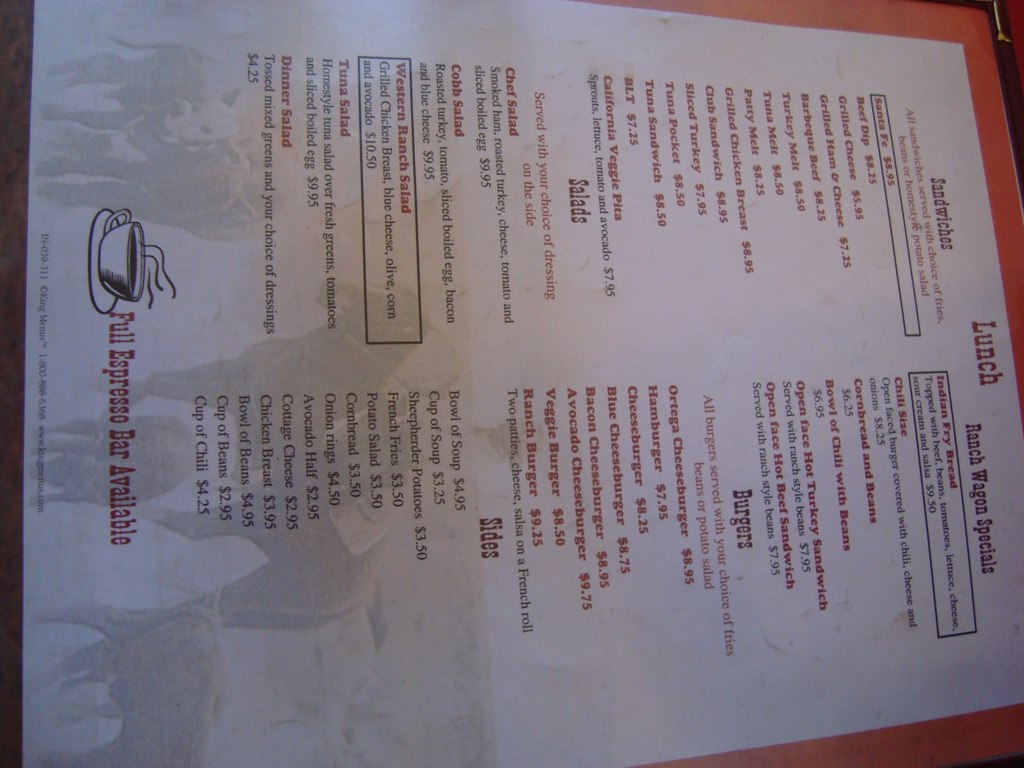The image showcases a lunch menu that is slightly tilted to the right. At the top of the menu, the word "LUNCH" is prominently displayed in red. The upper section, titled "Sandwiches," lists approximately 10 different types of sandwiches, each accompanied by their respective prices, also in red, though the text is somewhat out of focus. Below the sandwiches, there is a "Salads" section featuring options such as Chef Salad, Cobb Salad, Western Ranch Salad, Tuna Salad, and Dinner Salad.

Towards the bottom right corner, a section labeled "Ranch Wagon Specials" lists various items with their corresponding prices in black text. The subsequent section, "Burgers," also has items listed in red with prices next to them. Further down, there's a "Sides" section in red, followed by several items in black text, including a "Bowl of Soup."

At the very bottom of the menu, a black and white drawing of a coffee cup with steam rising from it is present, alongside the note "Full Espresso Available." The layout includes framed items and lines of tags that segment menu categories, enhancing its organized appearance despite the sideways orientation.